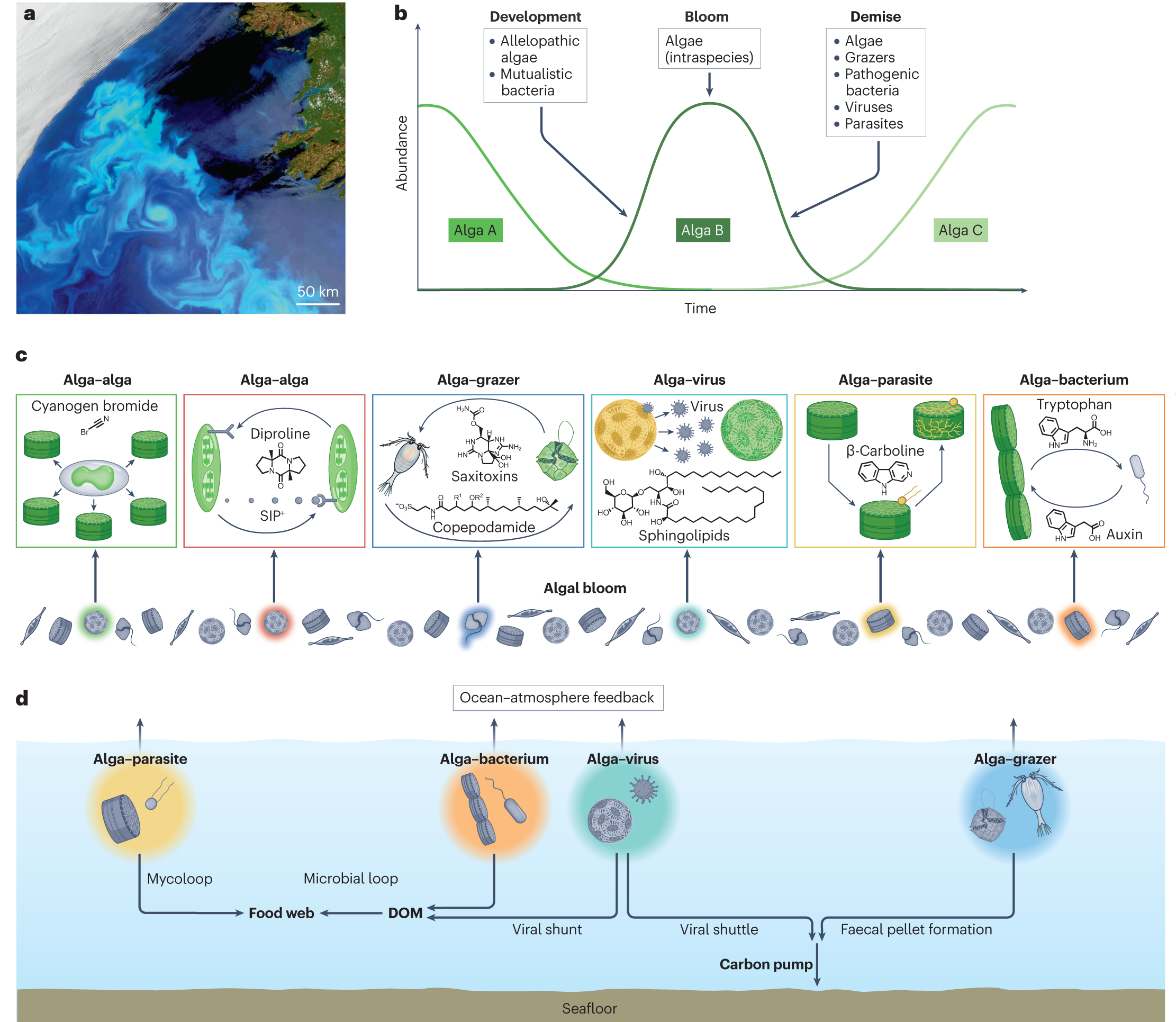This detailed infographic from a scientific magazine provides an extensive analysis of algae blooms and their ecological impacts. In the top left corner, an aerial image labeled "A" offers an overview of an oceanic region, showcasing the distribution of algae blooms with colorful blues and greens, and a 50 KM scale marker. Adjacent to it, a graph marked "B" illustrates the life cycle of algae blooms, charting different phases such as Development, Bloom, and Demise. The graph highlights various elements like allelopathic algae, mutualistic bacteria, bloom algae, algae grazers, pathogenic bacteria, viruses, and parasites.

Below these, images "C" and "D" delve deeper into the cellular processes and interactions at play. "C" features schematics of algae in different stages and the complex interactions between algae, grazers, ions, and other elements. "D" provides a comprehensive view of the ocean-atmosphere feedback loop, detailing the roles of algae parasites, the food web, the carbon pump, and entities like algae bacterium and algae virus, all the way down to the seafloor. This intricate diagram is set against a whitish background, segmented into various categories and interconnected lines, offering a thorough depiction of algae bloom dynamics and their environmental impacts.